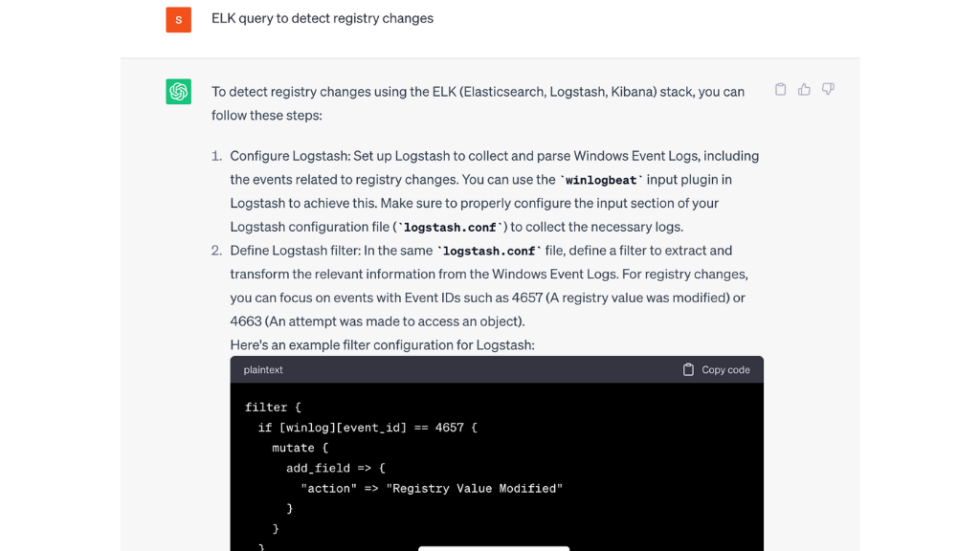Here we have an image illustrating a question posed to an AI program along with its response. At the top, in a white banner, there is an orange square with an 'S' icon asking the question: "ELK query to detect registry changes." Below, in a gray box, there is a green square icon displaying a spirograph-style image. This is followed by a detailed response explaining how to detect registry changes using the ELK stack (Elasticsearch, Logstash, and Kibana).

The response provides a step-by-step guide:

1. **Configure Logstash**: 
    - Set up Logstash to collect and parse Windows event logs, including events related to registry changes.
    - Use the `winlogbeat` input plugin in Logstash to achieve this.
    - Ensure proper configuration of the input section in the Logstash configuration file (`logstash.conf`) to collect the necessary logs.

2. **Define Logstash Filter**:
    - In the same `logstash.conf` file, define a filter to extract and transform relevant information from Windows event logs regarding registry changes.
    - Focus on events with specific event IDs, such as 4657 (a registry value was modified) or 4663 (an attempt was made to access an object).

An example configuration snippet for Logstash is provided, showing the filter setup:

```
filter {
  if [winlog][event_ID] == 4657 {
    mutate {
      add_field => {"action" => "registry value modified"}
    }
  }
}
```

The example is visually represented by a black image with the configuration details clearly formatted and easy to read.